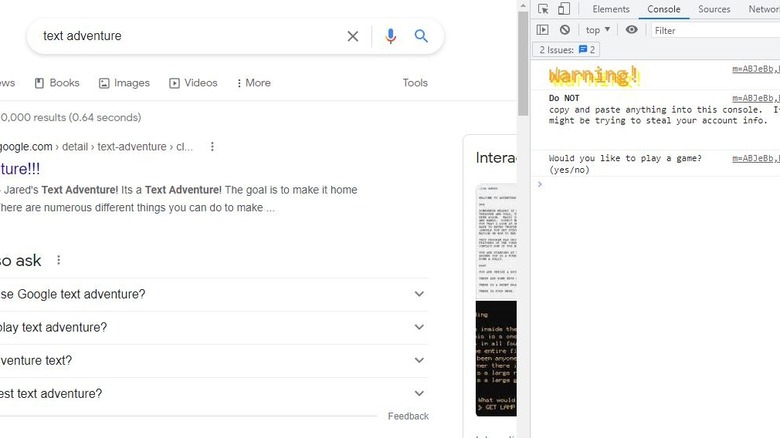This detailed caption accompanies a color image that appears to be taken from a web page. The image is divided into two main sections. On the right-hand side, there is a pull-up menu containing various tabs labeled "Elements," "Console," "Sources," and "Network." This section includes a filter option, currently showing two issues highlighted by yellow and orange warning signs with exclamation marks. A cautionary message reads, "Do not copy and paste anything in this console. I might be trying to steal your account info." Additionally, a text box asks, "Would you like to play a game, yes or no."

On the left-hand side, which displays the actual web page, the search box contains the query "text adventure." It took 0.64 seconds to generate the results, although zero results were found. The search appears to have been performed on google.com, detailing "Jared's Text Adventure." The text provides a brief description: "It's a text adventure. The goal is to make it home. There are numerous different things you can do to make it." Below this, there are additional clickable options and pull-down menus including "Google Text Adventure," "Play Text Adventure," "Adventure Text," and "Best Text Adventure." Finally, at the bottom right corner of the image, a "Feedback" option is visible.